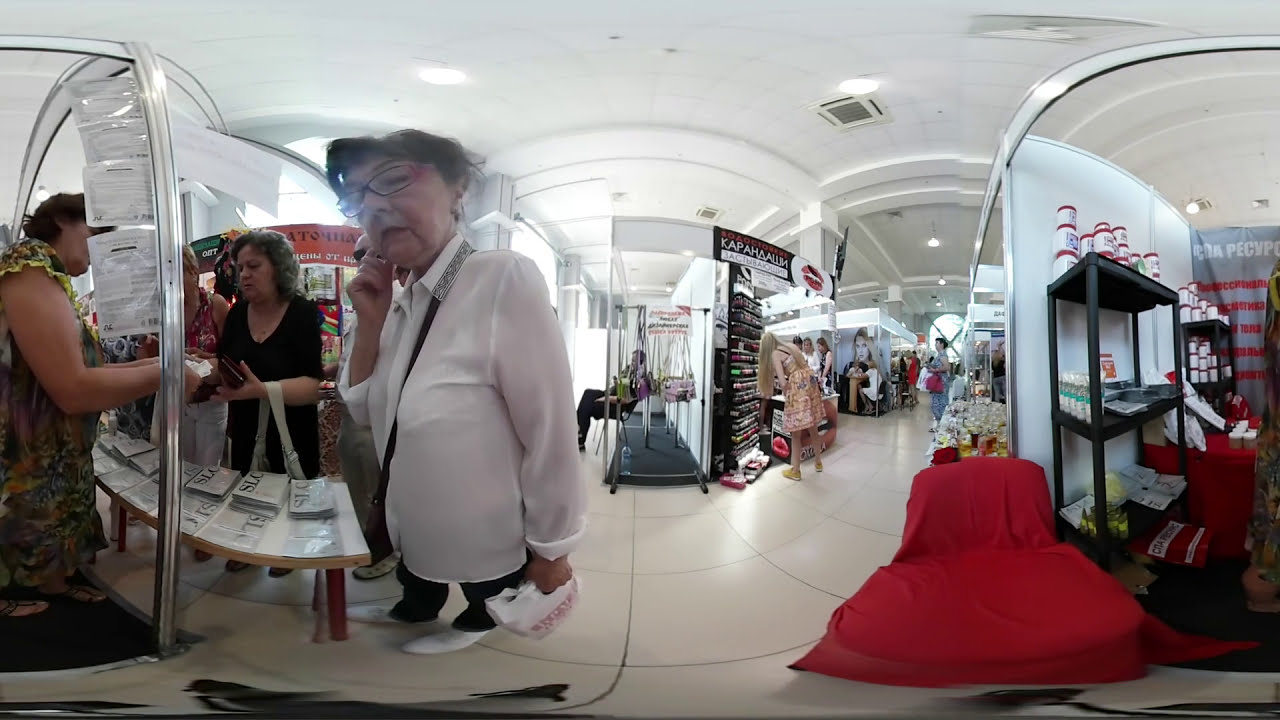In a bustling and slightly distorted scene within a shopping mall, an older woman with dark hair, wearing glasses and a white blouse, is prominently featured. She stands near the center of the image, picking at her right ear, her legs appearing unusually short due to a fishbowl distortion effect at the bottom of the picture. To her left, another woman in a black dress is engaged in a transaction with a third woman who is handing out pamphlets or possibly selling something. Further to the left, there is a woman in a colorful flower dress, likely yellow, green, and blue, appearing to sell or distribute something with words on it, potentially a book. 

On the right side of the image, a red chair is visible on the ground. Also toward the right, a woman in a white shirt, black pants, and white shoes, with a black strap across her chest, is holding a white bag. Behind her, a man in an all-black outfit sits with his legs crossed. Centered in the background, a woman with long blonde hair in a sundress, possibly yellow and white with black accents, is looking at makeup products, likely lipstick, suggested by a banner featuring lips above the stand. There are additional people in the busy background, shopping and moving through the mall, captured amongst white tiled floors and ceilings with integrated lights and speakers. Above the makeup stand is a black banner with white and red text, featuring a word that appears foreign, "Kapa'bamla."

The entire scene is lively, framed by white walls and shelves stocked with products, emphasizing a typical yet vibrant shopping experience.